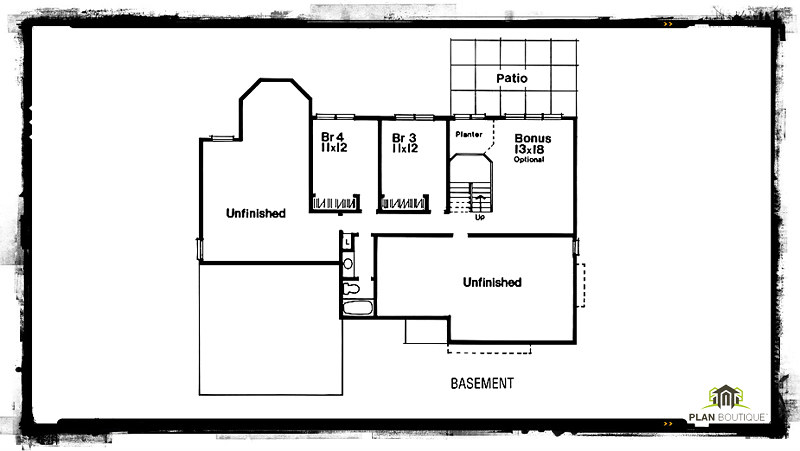The image depicts a detailed floor plan, possibly of a house. The outer perimeter of the plan has a dark, thick outline which appears smudged, giving it an uneven look. Within this boundary, there are various shapes representing different rooms, each carefully labeled.

Starting from the top-left corner:
- There is a partially drawn square with a unique diamond-shaped extension at the top labeled "unfinished".
- Directly below this, there's a black-outlined but blank square.
- Within the "unfinished" room, a line curves around to what seems to be a closet, labeled "BR4". The writing underneath "BR4" is too small to read.
- A continuation of this line leads to another closet marked "BR3", with similarly unreadable text beneath.

In the center-right of the plan:
- There's a dotted line indicating a window within a larger square shape. This area is labeled "Bonus 13x18", although the text under it is too small to decipher.

Above this section:
- A black-outlined rectangle, filled with vertical and horizontal lines, is labeled "Patio".

Further down the plan:
- A couple of partial squares curve around to form another area labeled "unfinished".
- Adjacent to this, an area that appears to be a bathroom.

Finally, the bottom section of the plan is marked "Basement".